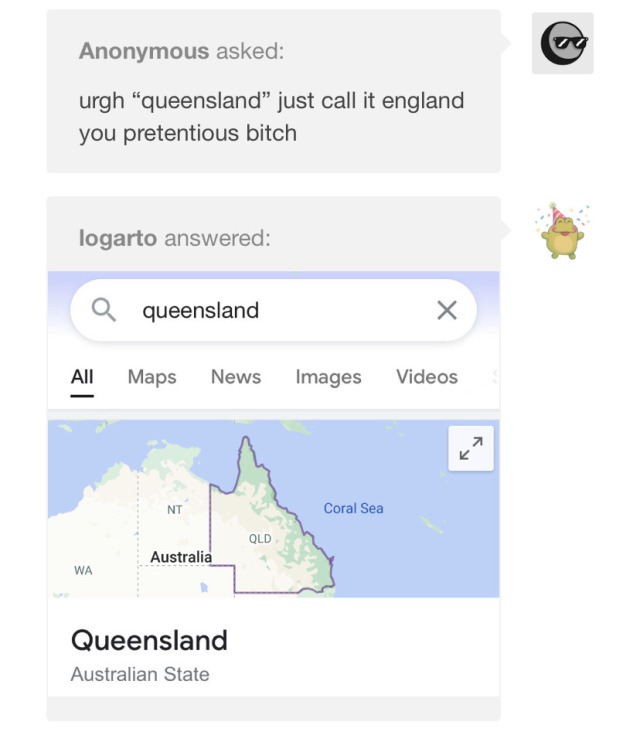In this image, at the top, there's text that reads "Anonymous asks," followed by a highlighted text in quotation marks: "you are gh Queensland." Below it, there's a response: "Just call it England you pretentious bitch." The message is presented on a gray background.

To the right, there's a light gray square profile picture resembling a wheel shape with sunglasses. Below the response, Lagordo answered "Queensland" as a Google search result, segmented into five categories: All, Maps, News, Images, and Videos.

A displayed map shows the region labeled as "Qld" with a purple outline. To the left of the map is Australia, and to the right is the Coral Sea. Below the map, "Queensland" is written in black text with "Australian state" in gray text underneath.

Lagordo's small profile picture, resembling a light brown animal with a party hat, is positioned beside the answer.

The detailed composition concludes here, providing a comprehensive description of the image from top to bottom.